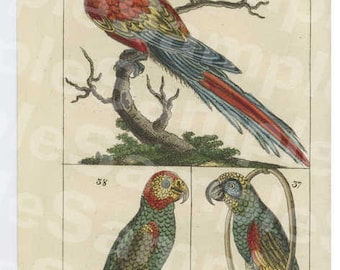This image is a detailed, vintage-style color illustration of parrots, likely segmented from educational or scientific material for children. The background has a sepia tone and features an illegible diagonal watermark, giving it an aged look. The illustration is in landscape format and showcases three main depictions of the parrots.

At the top, a large parrot is perched on a curved tree branch with green foliage. This parrot has a vibrant mix of colors: a red back, folded blue wings, and a tail with a combination of blue and red feathers.

Below this primary image, there are two smaller side-by-side illustrations. On the left, the parrot has a red head with a yellow outer border around the eyes, a green body, and wings that incorporate both red and green hues. On the right, the parrot features a light yellow head, a silver beak, a blue eye with a dark blue rim, and a body blending green, red, and yellow feathers. Each of these smaller illustrations is labeled with black numbers, 37 and 38, beside them.

The overall composition suggests the page is part of a larger book, textbook, or scientific document dedicated to the classification of birds, particularly parrots.